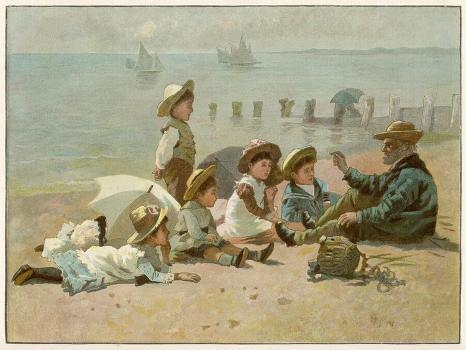The painting depicts a serene beach scene where an older man, dressed in a long-sleeved blue jacket and beige pants with a beige hat, sits on the sand. His knee is up and his arm is resting on it as he appears to be telling a story to five children. The children, dressed in old-fashioned clothing including wide-brimmed hats, are gathered around him; one stands, while the others sit or lie attentively. A sense of muted anticipation pervades the scene as they listen intently. In the backdrop, the remnants of a dock extend into the water, with a solitary figure holding an umbrella walking along it. Two distant sailboats add to the maritime atmosphere. The overall palette of pastel blues, beiges, and whites further lends a washed-out, vintage feel to the composition. A spilled basket lies next to the man, and a dog is spotted swimming nearby, reinforcing the idyllic and slightly nostalgic seaside setting.